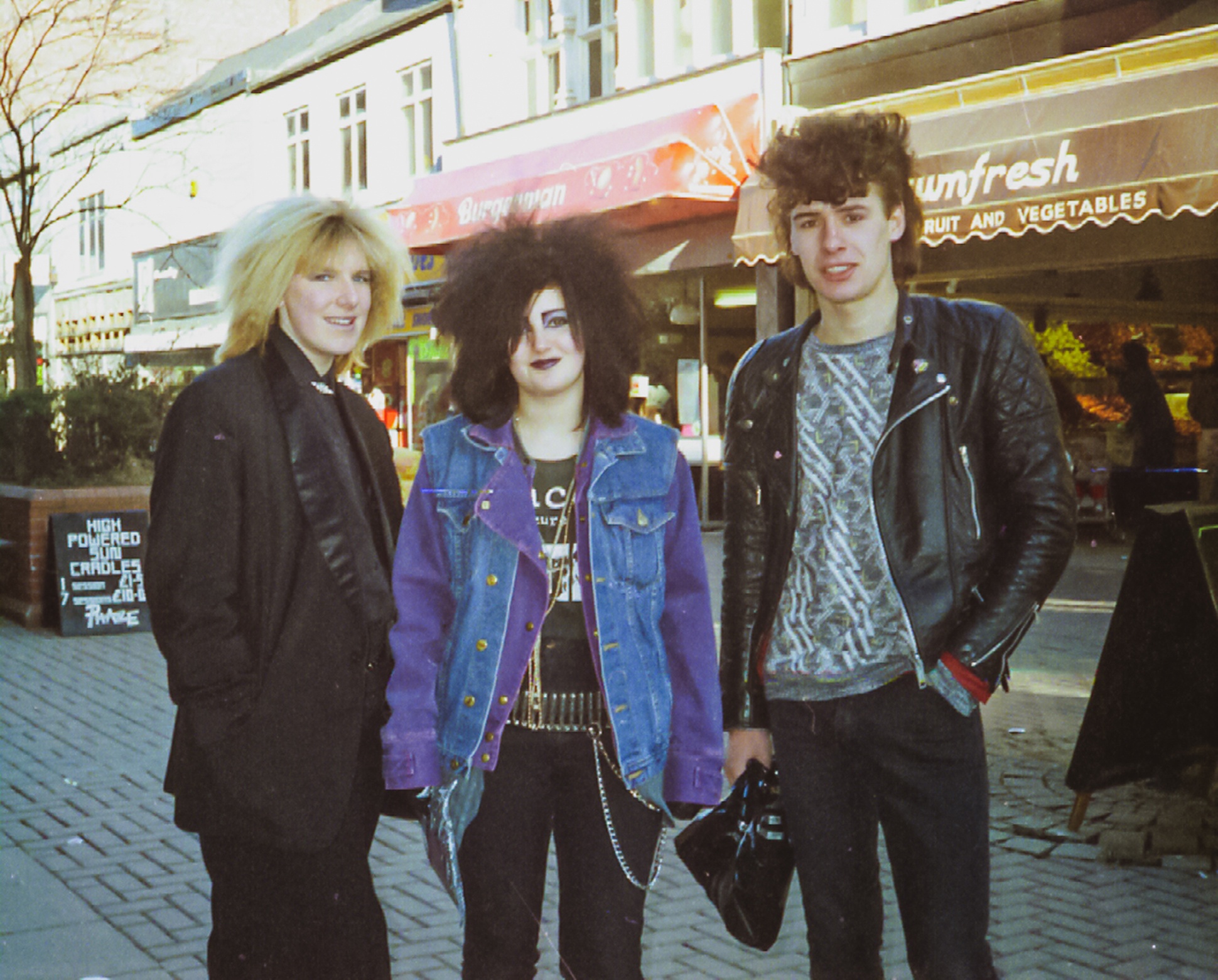In this vintage, slightly worn photograph, three youthful musicians exude a funky rock vibe as they stand on a brick-paved city street, surrounded by white buildings and storefronts. The vibrant street scene is dotted with awnings and displays, including a notable "Town Fresh Fruit and Vegetables" sign on the brown awning in the background, amidst other appealing grocery shops. On the left, a person with short, frizzy blonde hair reminiscent of Andy Warhol sports an all-black outfit, a tuxedo-style jacket with hands casually in the pockets, and smiles warmly. Their three-quarters profile reveals a Caucasian face with no makeup. In the center, a woman with frizzy, shoulder-length black hair and dark lipstick stands confidently in a purple and blue jean jacket, a black shirt with white print, black pants, and a silver belt with a chain hanging down her left leg. Completing the trio on the right, is a boy with short, dark curling hair, dark eyes and brows, who smiles broadly while dressed in a gray and white striped shirt under a black leather jacket, and black pants. A creative handbag accents his stylish appearance. The street buzzes with other people and vehicles in the background, enhancing the lively urban atmosphere of this captured moment.